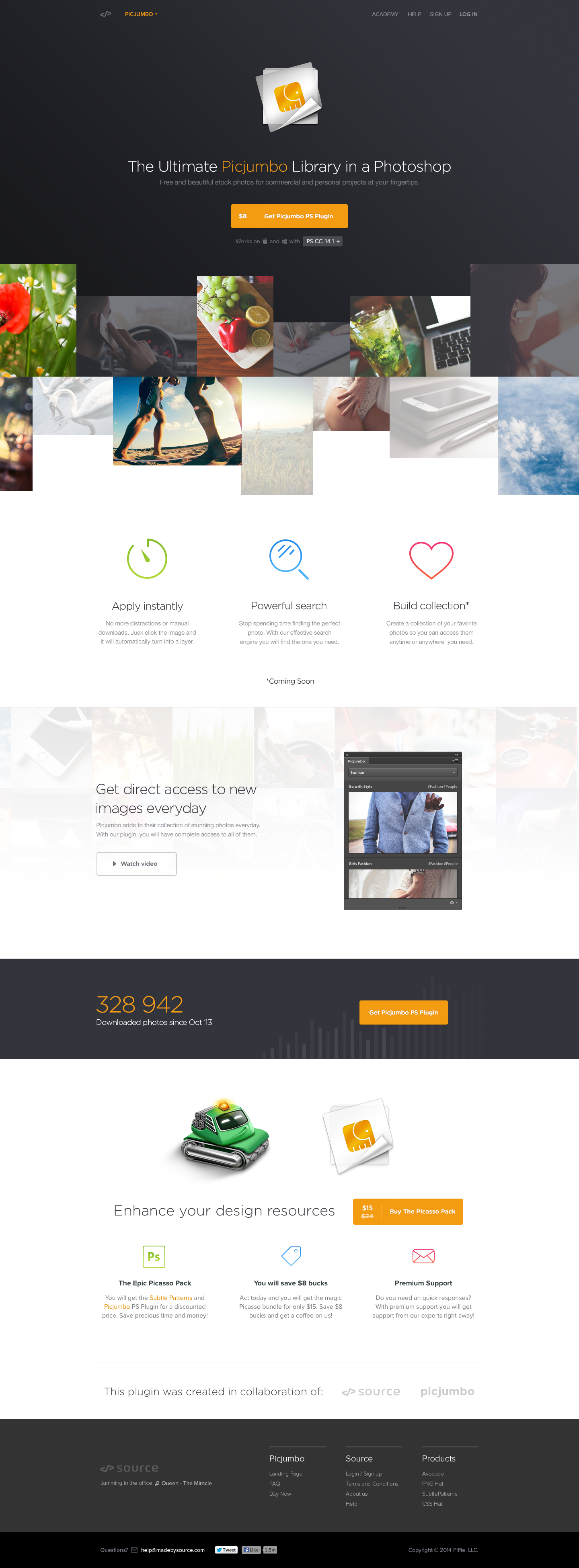This vertically oriented image is an advertisement for the Pick Jumbo Photoshop plugin. At the top of the image, set against a black background, the top-left corner features a small gray design accompanied by the text "Pick Jumbo" in vibrant orange. In the top-right corner, navigation options are listed in gray: "Academy," "Help," "Sign Up," and "Login."

Below this header sits a white paper icon adorned with an orange elephant drawing. Beneath the icon, the text reads, "The Ultimate Pick Jumbo Library in Photoshop." An orange button beneath this text encourages users to "Get the Pick Jumbo PS Plugin."

A variety of sample images are displayed, offering a preview of the diverse photos available. Icons with green, blue, and red themes feature key plugin benefits: "Apply Instantly" (with a green clock), "Powerful Search" (with a blue magnifying glass), and "Heart-filled Collection" marked as "Coming Soon" (with a red heart).

Further down, slightly faded images overlay more text, stating, "Get Direct Access to New Images Every Day," followed by more sample images and additional information. It reveals that "328,942 photos have been downloaded since October 13th" and includes another orange button to download the Pick Jumbo PS Plugin.

Towards the bottom of the image, additional benefits and offers are detailed, such as the "Epic Picasso Pack," a savings offer of $8, and a "Premium Support" button. The bottom section provides links to frequently asked questions, a "Buy Now" option, "About Us," "Help," and other product information.